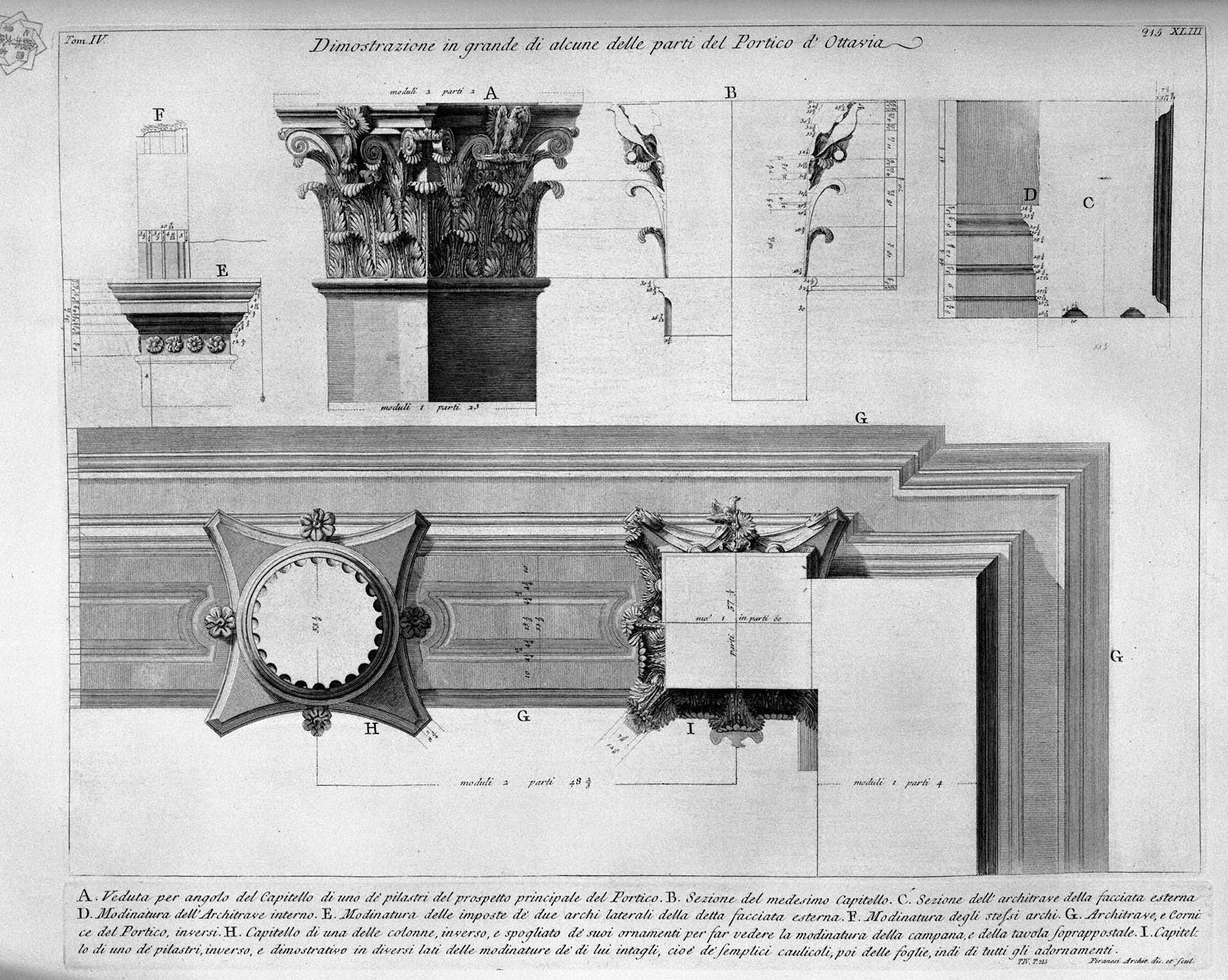The image is a black and white, grayscale sketch on paper, detailing an architectural blueprint of columns intended for construction. At the top, it features the title "Demonstrazione in grande di alcune delle parti del portico d'Octavia," likely indicating it is in Italian. The sketch meticulously showcases multiple views and intricate details of the columns, adorned with elaborate floral or leafy patterns. Various sections of the column are labeled with letters A through I. The overall image of the column is marked as A, while B shows a cross-section. Sections C, D, E, and F further detail different parts of the column, possibly depicting its shaft and base. G, H, and I illustrate what seems like door moldings or frames with G resembling a door frame overlayed by a square mechanism with points. Roman numerals adorn the top edges of the sketch, adding to its antiquated and precise presentation. Overall, the sketch is an exquisitely detailed, fine-lined architectural drawing, presenting both side and top views of the column elements alongside descriptive text primarily in Italian or Latin.